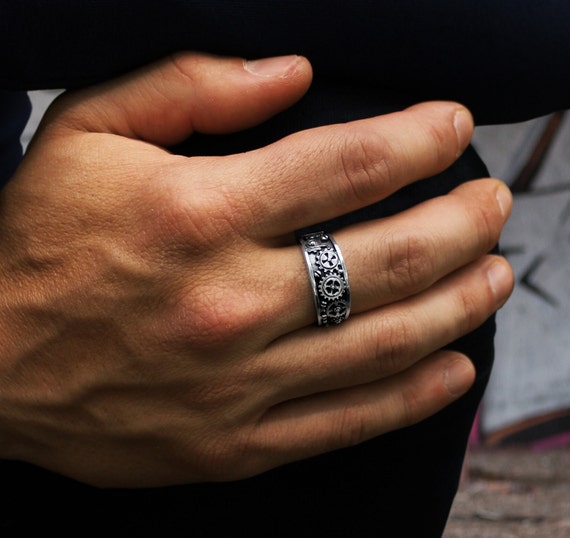In this detailed close-up photograph, the primary focus is on the well-manicured right hand of a white man, possibly in his 20s to 40s, showcasing an intricate silver ring on his middle finger. The ring, made of what appears to be titanium or stainless steel, features a distinctive steampunk design, adorned with numerous stylized gears welded together to create a metallic, mechanical aesthetic. The man's hand, which is notably veiny, seems to be resting on a surface that could either be his knee covered in black pants or a black velvet fabric, presenting a formal and sophisticated appearance. The background of the image is blurred, revealing vague elements like a gray object, potentially a book, and a dark brown, striped floor, without any visible artist trademarks or text. This photograph appears to be an advertisement or a display of a unique piece of jewelry, emphasizing the ring's detailed craftsmanship and artistic flair.